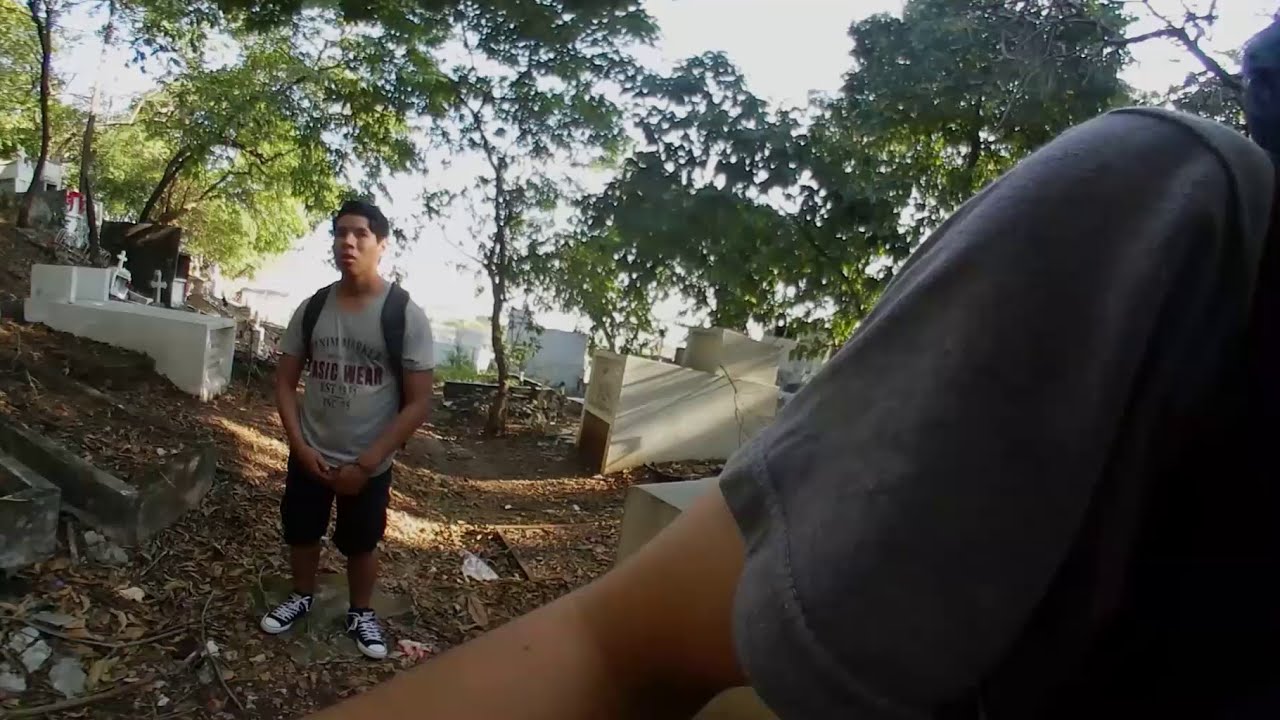In the image, there is a young man standing slightly to the left, appearing both startled and contemplative. He sports a backpack and is dressed in a gray t-shirt with the words "basic wear" or "AFIC Wear" visible, black shorts, and black and white Converse shoes. His short black hair and light brown complexion are noticeable. The setting is an old graveyard with brown fallen leaves scattered on the ground, giving it a somewhat neglected appearance. Tombstones with white crosses punctuate the scene, which features hilly areas flanked by large rectangular plots. Green trees, covering much of the overcast but bright sky, form the background. On the right-hand side, a partial figure—likely another man—clad in a dark blue, short-sleeved t-shirt and also of light brown complexion, is visible. The scene captures a moment full of ambiguity, leaving one to wonder if the individuals are paying respects or involved in something unexpected.